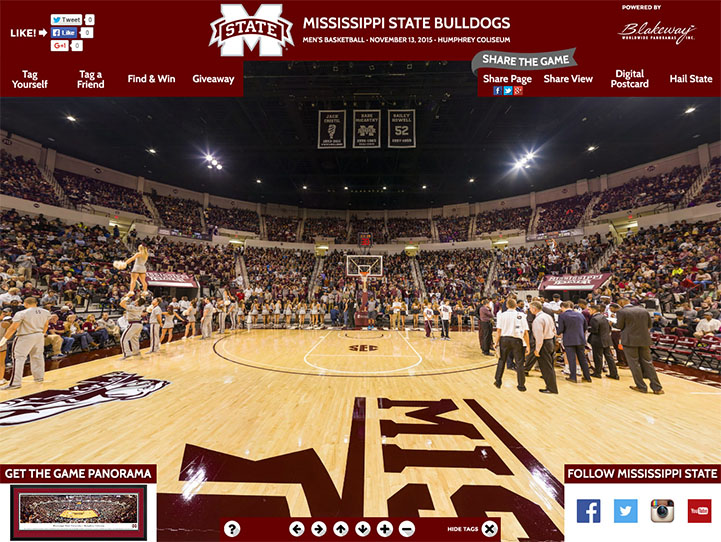**Caption:** 

A vibrant scene from the Mississippi State Bulldogs Men's Basketball game against Michigan State on November 13, 2015, at the Humphrey Coliseum. The panoramic view spans from one side of the court to the other, filled with enthusiastic fans. Cheerleaders are seen energizing the crowd on the left side, while on the right, a group of men in suits gather, possibly team officials or media personnel. The light wood floor features prominent Michigan State logos. The top of the image displays the game's title along with the Michigan State logo and a "powered by Blackway" note. To the left, various social media and interaction options are available, including liking the picture on Twitter and Facebook, tagging friends, and entering giveaways. The right side offers sharing options like digital postcards and "Hail State" messages. In the bottom corners, there are additional features promoting social media engagement, with logos for Facebook, Twitter, Instagram, and YouTube.